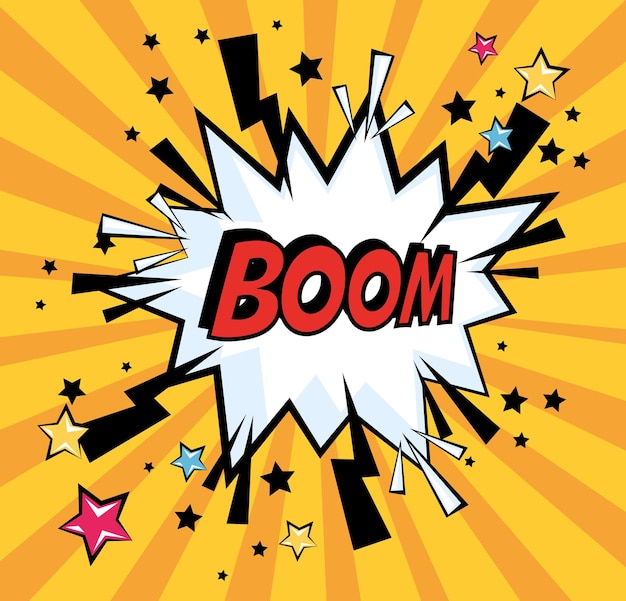This square image is a vibrant cartoon explosion with a comic book flair. At the center, a jagged, starburst-like shape outlined in black is filled with stark white. Bold red letters spelling "BOOM," outlined in black with a 3D drop shadow effect, dominate the middle. Black lightning bolts radiate outward from the white center, reaching almost to the word "BOOM". Surrounding this central burst are various stars—some black and others in red, yellow, blue, and pink—along with smaller black dots. The background features a dynamic sunburst pattern in yellow and orange, with alternating stripes extending to the edges of the image, adding to the explosive energy.